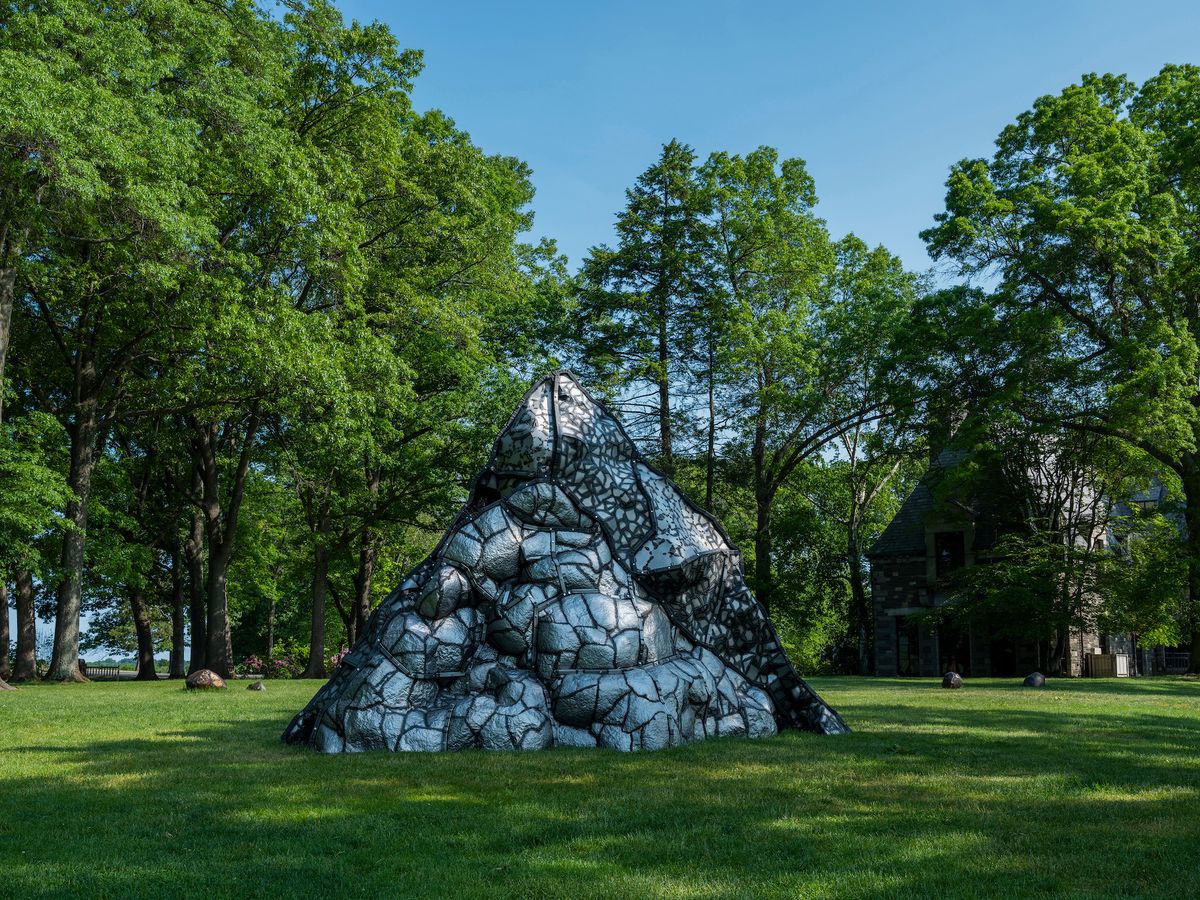This photograph captures a serene park setting on a beautiful sunny day. The sky is a clear blue, providing a striking backdrop to the lush greenery below. A row of large deciduous trees, with their vibrant green leaves, lines the background. Among these trees, partially hidden, is a two-story stone building with a tall peaked roof that could be either a church or a cabin-like house.

In the forefront, centered on a broad expanse of flat, green grass, stands a large, abstract outdoor sculpture. This striking public art piece is pyramid-shaped and appears to be constructed from numerous rocks of varying shapes and sizes, intricately fitted together. The structure is predominantly gray and black, with a texture that resembles a spider web design running through it. The sculpture, smooth yet jagged in appearance, rises to about a third of the height of the surrounding trees, making it a significant and imposing feature of the landscape.